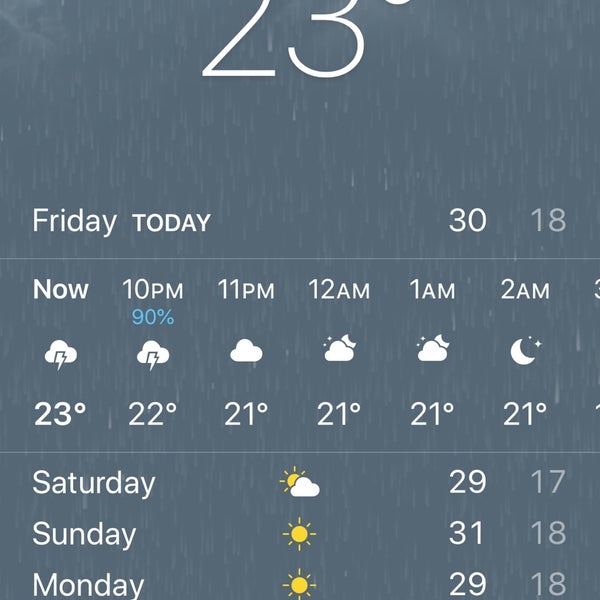The image is a screenshot captured from a weather application on a smartphone. The top section of the screenshot features a gray background with raindrop patterns, possibly indicating rainy conditions. The temperature display appears to be partially cut off, but it shows a reading of "23" degrees. Below this background, there's a detailed weather summary for the current and upcoming hours as well as days.

In the middle-left of the screen, the day is specified as "Friday," labeled as "today." The temperature forecast for the day indicates a high of 30 degrees, displayed in white, and a low of 18 degrees, displayed in gray.

Running vertically down the middle of the screen is a time-stamped forecast banner providing hourly weather updates:
- **Now**: Thunderstorms, 23 degrees
- **10 p.m.**: 90% chance of thunderstorms, 22 degrees
- **11 p.m.**: Cloudy, 21 degrees
- **12 a.m.**: Partly cloudy, 21 degrees
- **1 a.m.**: Partly cloudy, 21 degrees
- **2 a.m.**: Clear skies with a moon and stars icon, 21 degrees

At the bottom of the screen, a three-day weather forecast is presented:
- **Saturday**: Partly sunny with a high of 29 degrees and a low of 17 degrees
- **Sunday** (not Monday as duplicated in original): Sunny with a high of 31 degrees and a low of 18 degrees
- **Monday**: Sunny with a predicted high of 29 degrees and a low of 18 degrees

This comprehensive weather summary provides a clear overview of the anticipated weather conditions over the next several days, along with detailed hourly forecasts for the current night.